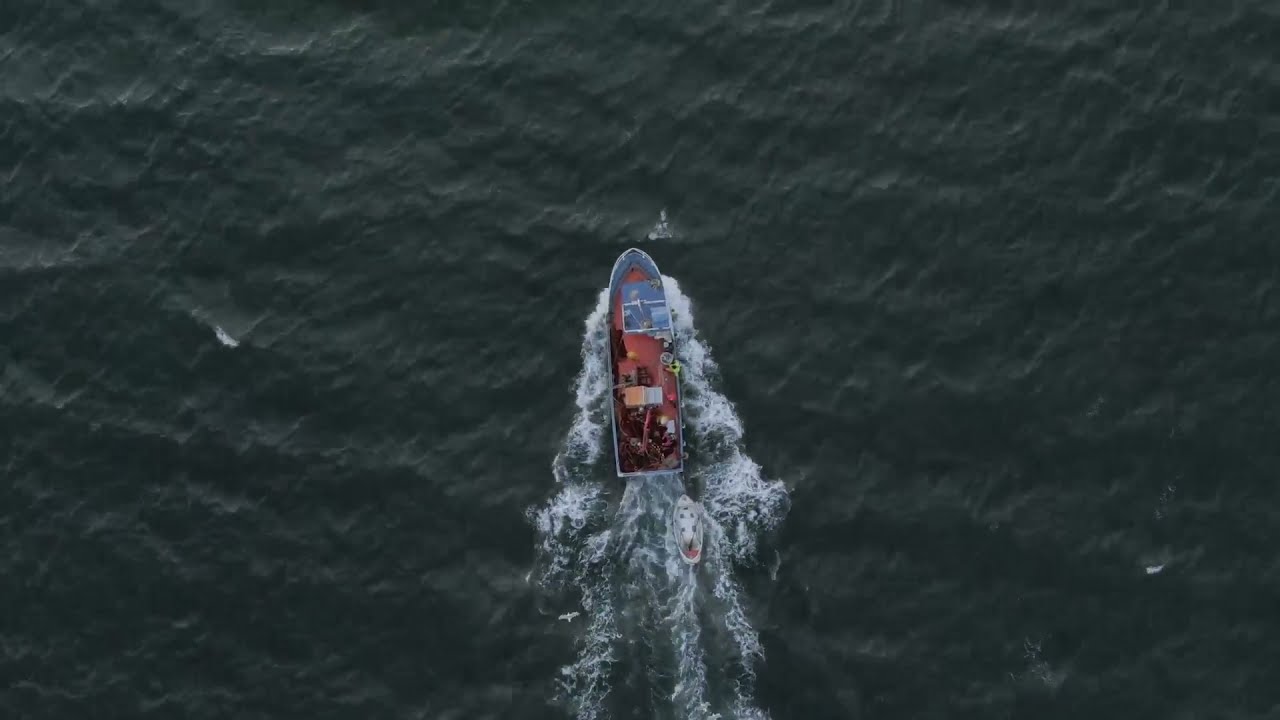In this aerial view photograph, a motorized fisherman's sailboat, characterized by a mainly light brown body with a gray covering at the front, cuts through a greenish-gray ocean, creating visible white streaks in the water that suggest its fast movement. Trailing behind and to its right is a smaller raft-like boat, also part of the scene. The boat's interior features various boxes, likely containing fishing equipment or other gear. The sea around the boats appears choppy, with small waves indicating a breezy journey. There are no visible people onboard, and the vast background is dominated by the expansive, slightly turbulent greenish-gray ocean.